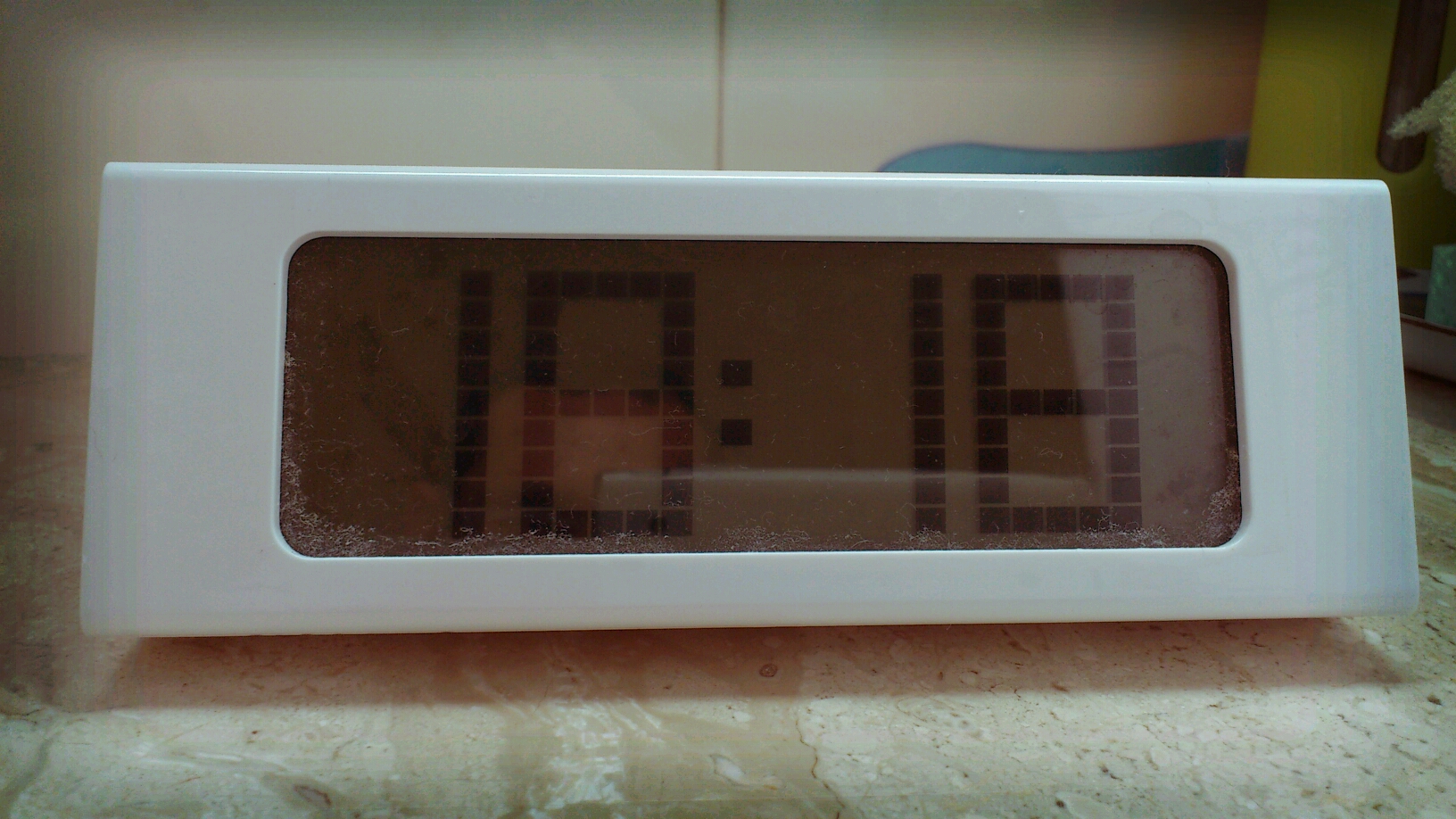This image depicts a rectangular digital clock displaying the military time 18:18. The clock features a white casing with a slightly tinted gray, clear screen that presents blocky black numbers. It appears somewhat dated in design and functionality and isn't plugged in. The clock is positioned on a worn and chipped concrete surface revealing a darker shade beneath, suggesting age or neglect. The background includes a slightly stained counter that adds to the overall impression of an infrequently used space. Additionally, the surrounding environment includes a tan wall, some yellow and blue objects in the corner, and what looks to be folding doors, possibly indicating the setting as a bathroom with artificial lighting.